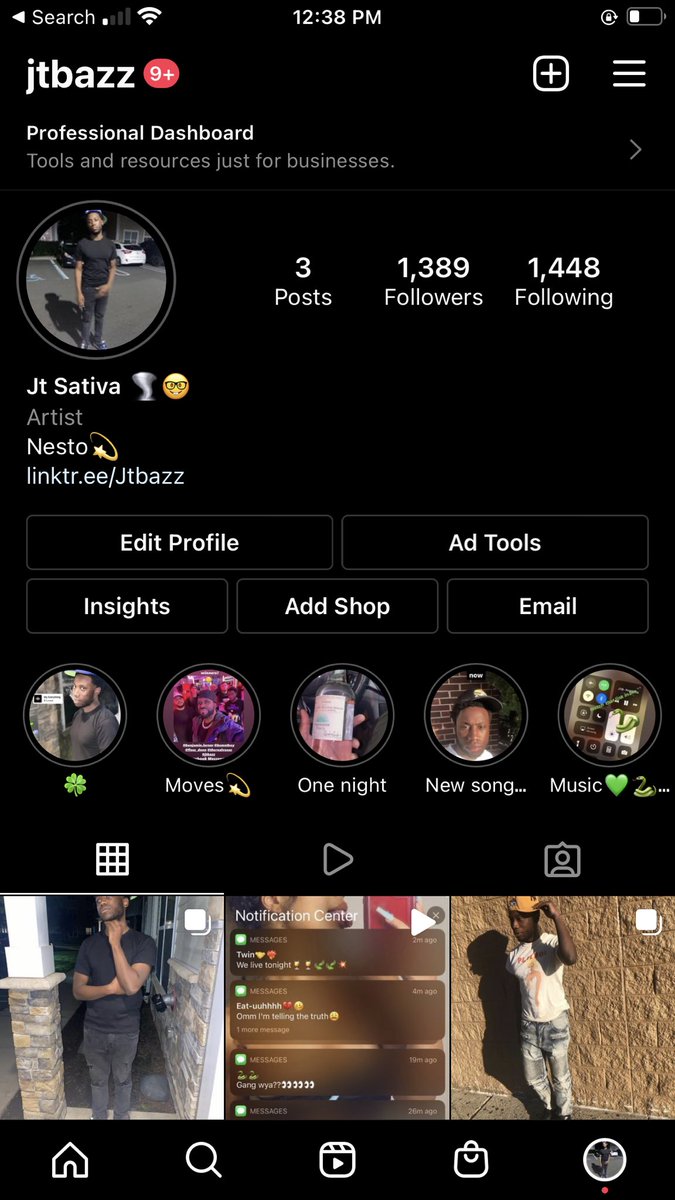This is a detailed screenshot of an Instagram profile viewed in dark mode. The background is black, and the text appears in white. At the top, there is a back button and the word "Search," indicating that a user search was performed. The time displayed is 12:38 p.m., and the phone's battery is at approximately one-third capacity. 

The user being viewed is "JT Sativa," with the username "JTBAZZ." There's a red notification bubble with a white "9+" indicating messages or notifications. Below the username, it says "Professional dashboard tools and resources just for businesses." 

The profile picture shows a Black male in his 20s or 30s standing in a dimly lit parking lot, wearing a black shirt and dark gray or dark blue pants. JT Sativa has made three posts, has 1,389 followers, and is following 1,448 accounts. His profile includes a tornado emoji and a nerdy smiley face emoji with glasses. He describes himself as an "artist" and "Nestro," followed by a star emoji. The bio contains a Linktree link: "linktr.ee/jtbazz."

At the top of the profile, there are standard action buttons including "Edit Profile," "Add Tools," "Insights," "Add Shop," and "Email." There are also story highlights below the bio section. At the bottom, three of his posts are visible, displaying various photos he has shared.